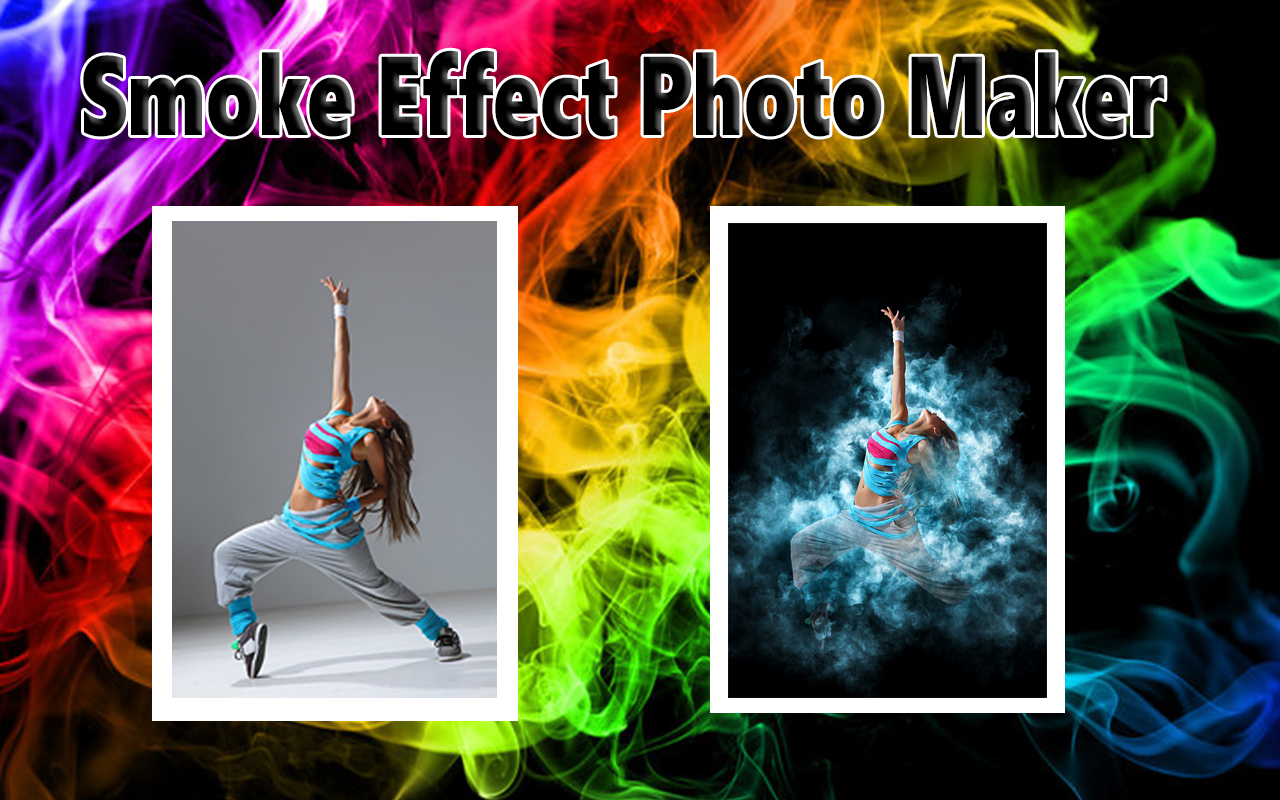The image features a dynamic presentation showcasing the capabilities of a smoke effect photo editing tool. At the top, bold white-outlined text reads "Smoke Effect Photo Maker," set against a vivid black background. The entire background is filled with swirling, rainbow-colored smoke, with hues of blue, purple, red, orange, yellow, and green transitioning smoothly across the image.

Centrally, two photographs of a woman in a dancing pose are displayed side by side in portrait orientation. The woman, dressed in a pink top adorned with blue ribbons that extend down to her waist, paired with gray sweatpants, and white and black sneakers, is caught in a poised, lunging position with one arm extended upward. In the left photo, she stands on a white floor against a gray background, exuding energy and motion. In contrast, the right photo transforms dramatically—surrounding her with a dynamic white and blue smoke effect that makes it appear as though she is suspended in an ethereal, turquoise mist, all set against an entirely black background, including the floor.

This visually rich graphic design showcases the transformative power of the smoke effect, blending realistic photography with striking special effects and typography. It not only highlights the tool's functionality but also emphasizes the dramatic changes possible with its use.